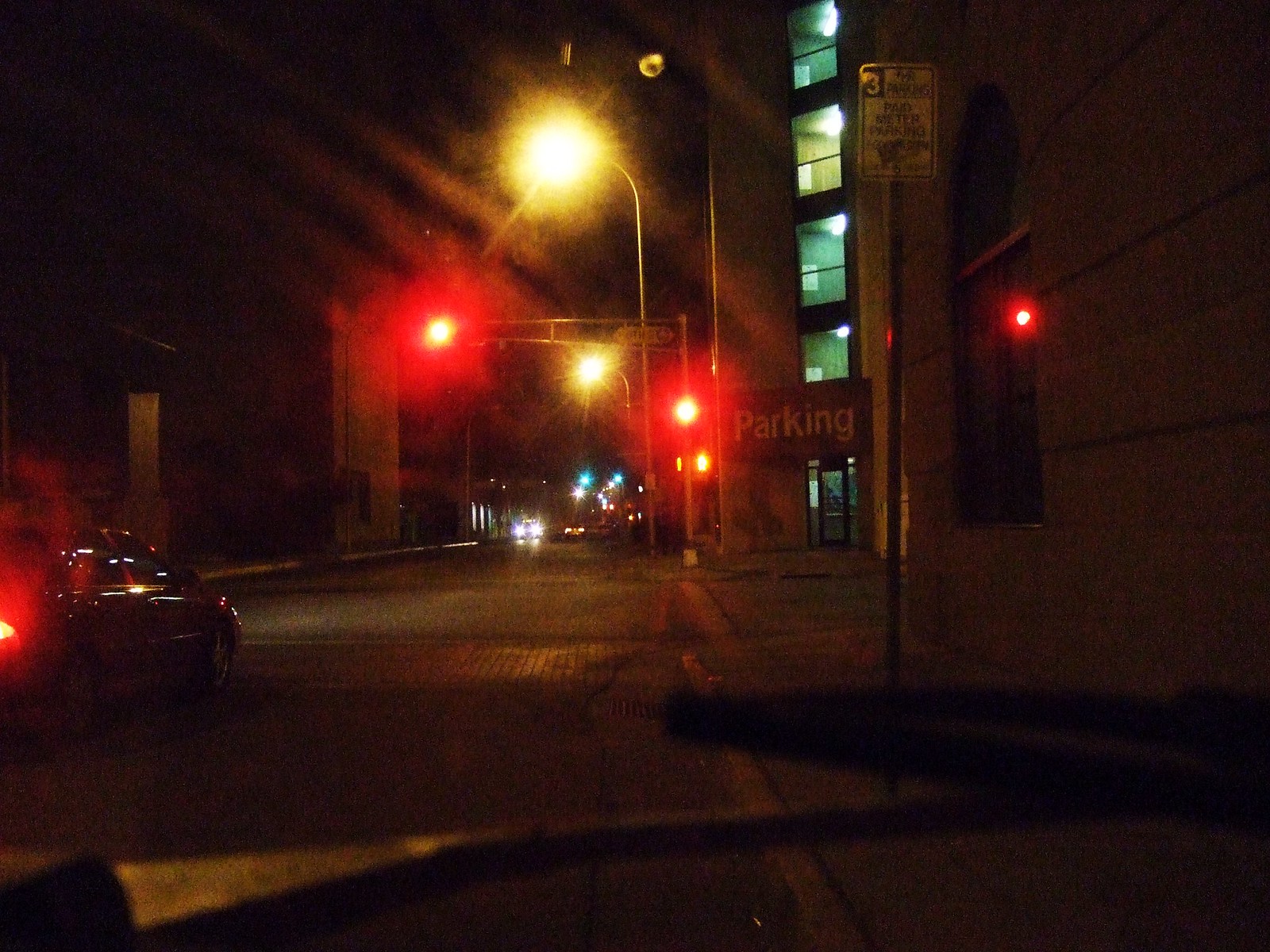This nighttime cityscape captures a bustling street illuminated by a towering streetlight arching overhead. A multi-level parking garage stands prominently, its lower floors displaying a mix of green and gold hues through rows of windows, with a door visible at street level. Three traffic lights, all glowing red, regulate traffic flow — one dedicated to a side street and two overseeing the main thoroughfare. Vehicles populate the scene, including a car and a truck heading towards the camera while another car recedes into the distance. The street itself is paved with bricks, adding a touch of classic urban charm to the vibrant scene.